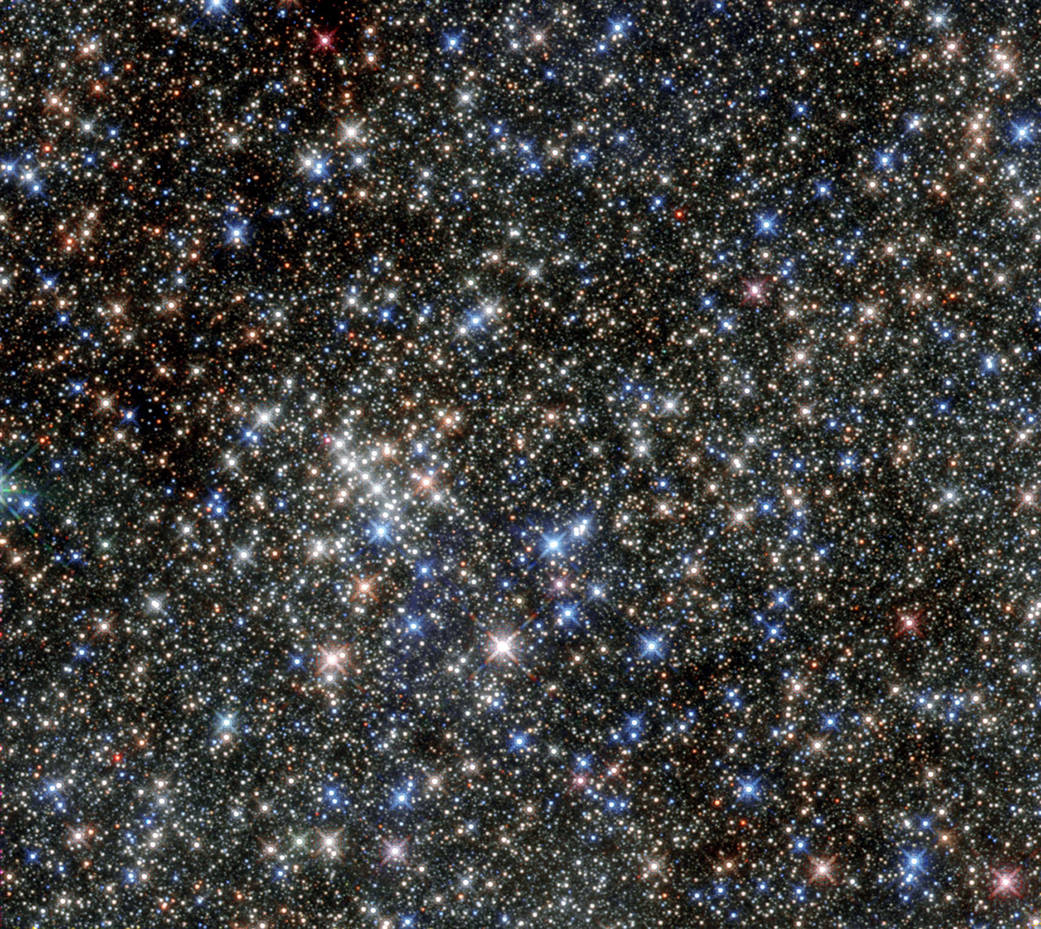The image showcases a breathtakingly starry night sky, dominated by a deep black backdrop teeming with thousands of twinkling stars. The stars, which appear as white dots, are accompanied by variously colored lights including blues, pinks, oranges, reds, and yellows, casting a vibrant, almost surreal glow. These celestial points of light vary in brightness and are dispersed across the sky, evoking the sense that the image was captured through a powerful telescope. The scene vividly portrays the majesty of the cosmos, capturing the myriad hues and intensities of the stars against the infinite blackness of space.